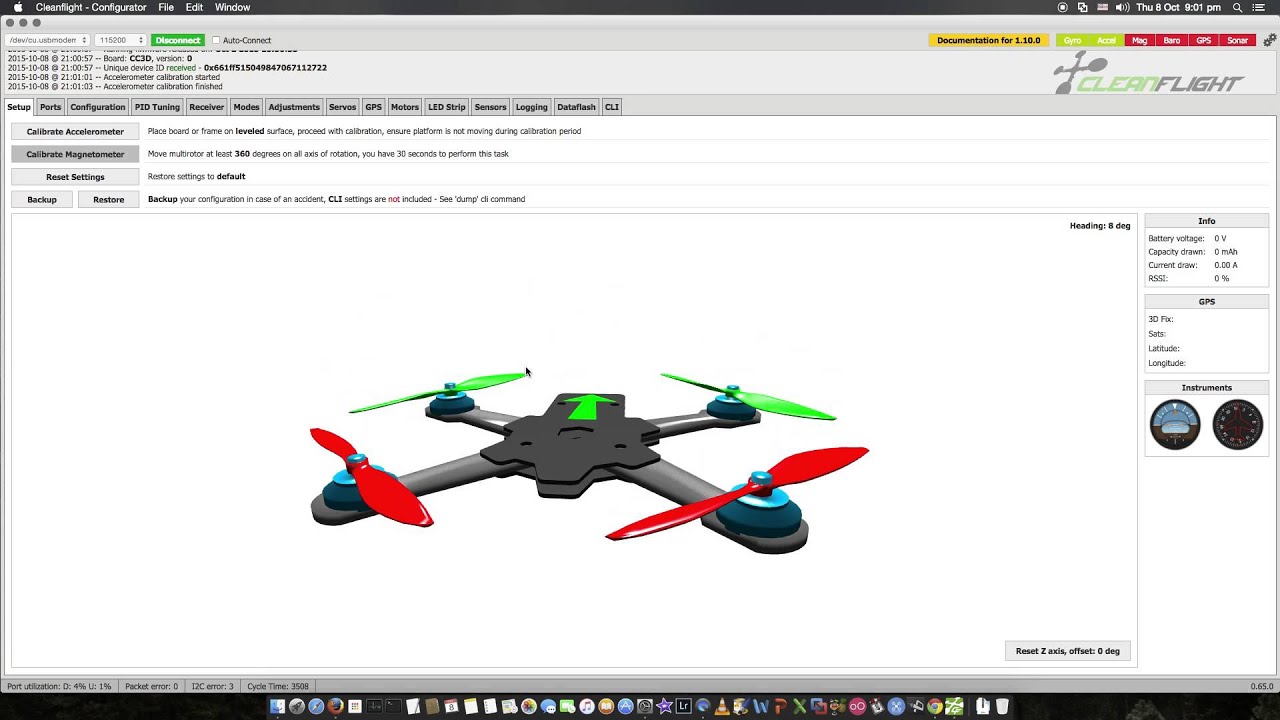Screenshot of a Clean Flight Drone Web Page on an Apple Device

This image is a screenshot taken on an Apple device, displaying a webpage mostly in white with subtle gray tones. At the very top, a dark gray bar includes the distinctive white Apple logo, alongside options for "File," "Edit," and "Withdraw." The system clock reads Thursday, October 11th at 9:01 PM. Just below this, a search bar allows users to navigate the site.

The central focus of the webpage is the Clean Flight drone platform. The Clean Flight logo, featuring a drone graphic, stands prominently, with "Clean" in green text and "Flight" in gray. Below the logo, several navigation tabs are visible, including "Setup," "Parts," "Configuration," "Tuning," "Receiver," "Modes," "Readjustments," "Screws," "CFS," "LED Strip," "Logging," and "CLT." These tabs suggest comprehensive options for drone customization and monitoring.

An illustration of a drone is also present, characterized by its gray and black body, red and green propellers, and blue accents, embodying a sleek and modern design. Additionally, there appears to be a time-tracking feature at the top of the page, adding to the operational insights provided by the site. Overall, this screenshot captures a detailed interface for drone enthusiasts and professionals looking to configure and optimize their UAVs.